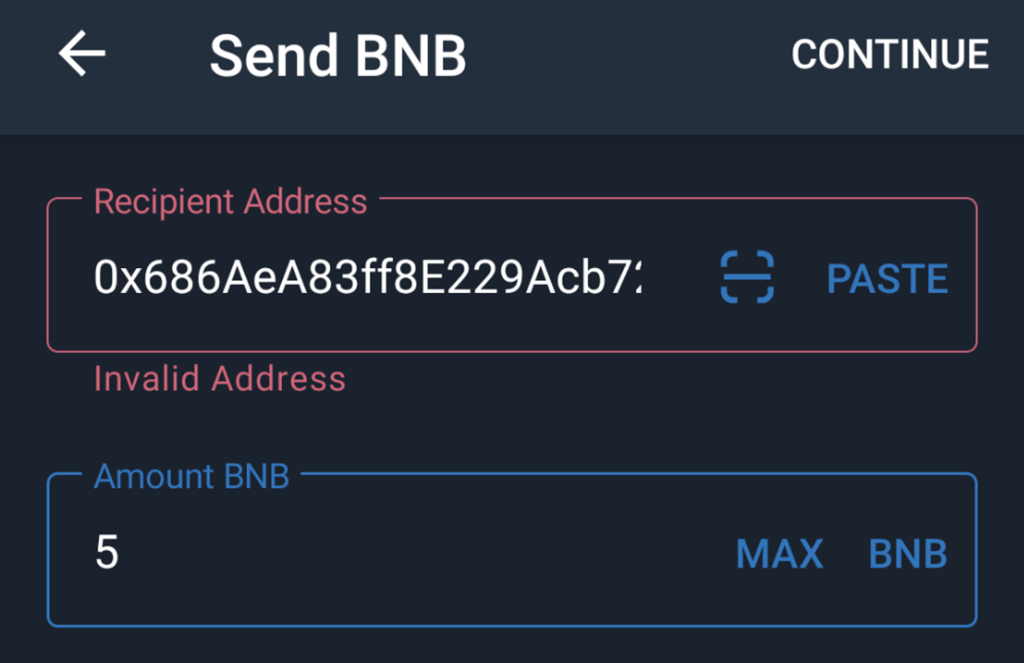**Image Description: Cryptocurrency Transaction Interface with Error Notification**

The interface has a sleek black background. At the top, a long charcoal gray rectangle extends across the width, featuring white text. On the left side of this rectangle, there is a directional arrow pointing to the left, followed by the text "send BNB," where "BNB" is capitalized. To the far right of this rectangle, the word "continue" appears in white text.

Below this, a long rectangle outlined in red is displayed prominently against the black background. In the top left corner of this red-outlined rectangle, the text "recipient address" is shown in red. Directly beneath this, in white text, is the partially obscured address "0x686AEA83FF8E229ACB7...", accompanied by a small blue square with rounded corners and a line through the middle. Beside this blue square, the word "PASTE" is written in blue, capitalized text. Below the recipient address, a red text notification reads "invalid address," indicating an issue with the provided address.

Further down, there is a long blue rectangle, outlined in the same blue. In the top left corner of this blue-outlined rectangle, the text "amount BNB" appears in blue, with "BNB" capitalized. Beneath this label, the number "5" is displayed in white text. To the far right within the blue-outlined rectangle, the word "MAX" is written in blue capitalized text, followed by "BNB," also in blue capitalized text.